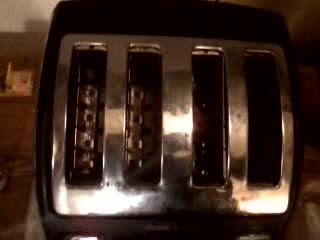The image depicts a very low-quality, low-resolution colour photo of the top of a black toaster, taken from a top-down angle. The toaster features four vertically-oriented slots, split into two pairs, with the left pair partially illuminated, and the right pair cast in shadow. The illumination suggests the use of a flash that only reached the left side. Surrounding the slots is a shiny, stainless steel trim, which is highly reflective, showing faint images of a kitchen in the background including cupboards, a countertop, and possibly a lamp. The photo is closely cropped, cutting off parts of the toaster at the bottom and top, while the left side reveals a hint of a wooden countertop beneath. Detailed, yet obscured reflections on the stainless steel include the outline of the photographer's head and shoulders, partially visible due to the reflective surface. The overall setting appears to be a dimly lit kitchen, contributing to the shadows and limited visibility in the image.